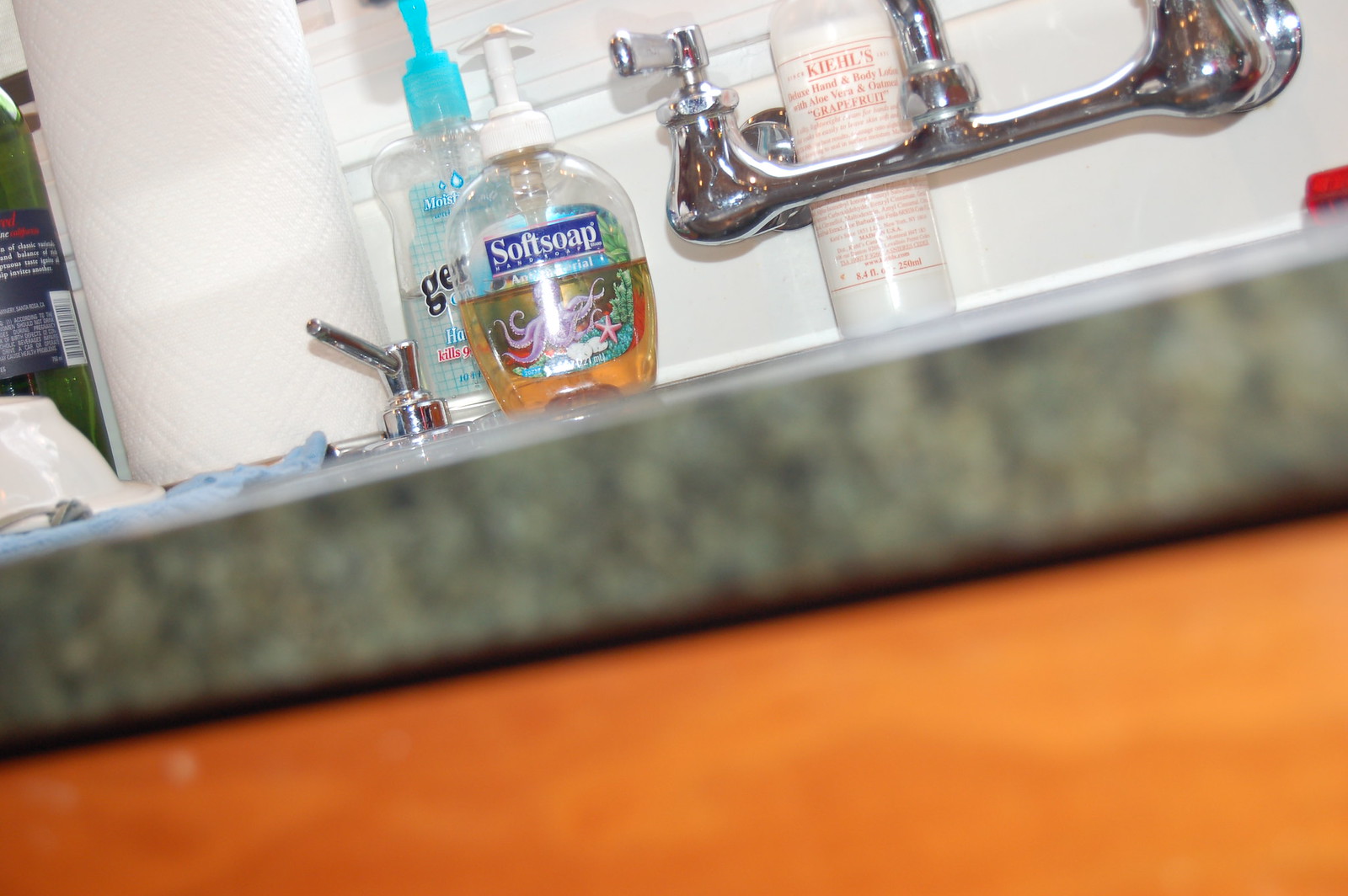In this intriguing photograph, the countertop, potentially part of a kitchen or bathroom, is captured with a noticeable slant. The surface features a striking pattern composed of gray, black, and white hues, running primarily from left to right. Prominently displayed is a portion of the sink, including the left-hand dial designed as a paddle switch, along with a built-in stainless steel soap dispenser situated to the left of the faucet.

Adjacent to the soap dispenser is a neatly stacked roll of paper towels, wound tightly. Positioned in front, there is an upside-down bowl placed atop a rag, suggesting it is drip-drying. Just behind the soap dispenser, a Germ-X hand sanitizer bottle with an aqua blue pump is visible, about half-empty. In front of this, a half-full bottle of Softsoap features a playful design of an octopus and a starfish, enclosed in an orange pump bottle with a dark blue and white logo.

Further behind the sink, a bottle of Kiehl's hand and body lotion stands almost three-quarters full. This white bottle, adorned with orange text, specifies its contents as aloe vera and oatmeal-infused, grapefruit-scented lotion. On the right side of the sink, there is a small red sponge or cloth. The bottom portion of the image predominantly showcases the brown cabinetry beneath the countertop.